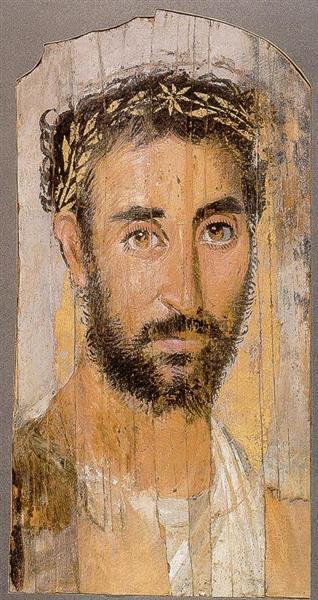This image depicts a Renaissance-style portrait, painted on a slightly worn, grayish-brown wooden board shaped reminiscent of a headstone. The painting features a tan-skinned, olive-toned man with thick black hair, arranged in short, slightly curly or wavy fashion. He sports a scruffy beard and mustache that connects from his sideburns around his chin, and thick black eyebrows above his expressive, bright brown eyes. A crown of golden laurel leaves adorns his forehead, suggesting a classical or historical influence, perhaps evoking Greek or Biblical times. He appears pensive, gazing directly at the viewer with his lashes highlighting his large eyes. The man's attire includes a semi-sheer, white garment through which his skin tone is faintly visible, hinting at a robe or shirt. The painting medium suggests it may have been created using acrylic or oil, adding to its classical aura and contributing to the worn effect, suggesting it has been preserved over centuries.